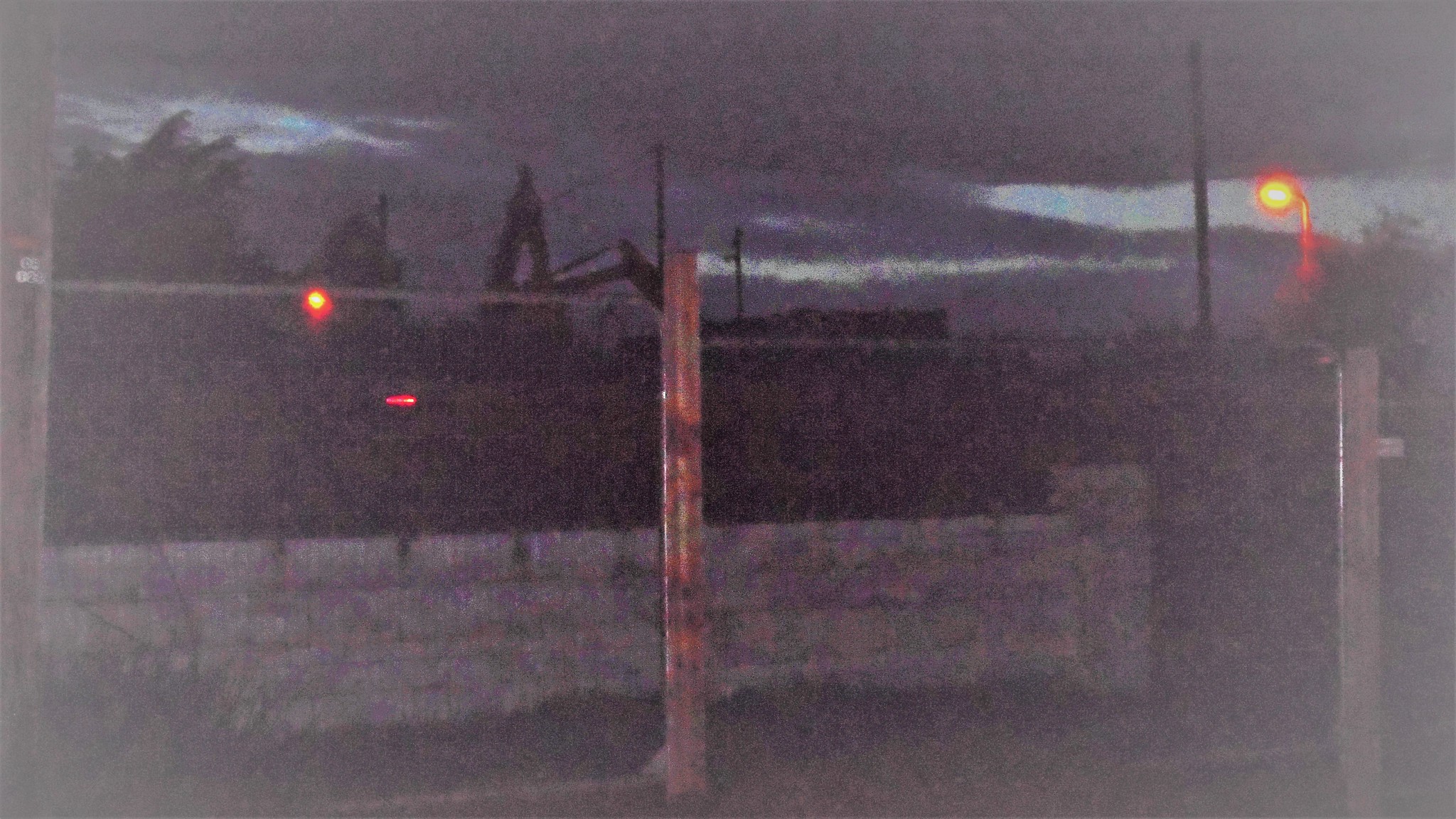The grainy image, taken at dusk, captures a dimly-lit outdoor setting with a slightly bright but darkening sky dotted with dark grey clouds. Dominating the foreground is a grey stone or brick wall, which appears to have another structure or wall rising higher behind it. Various lights illuminate the scene; some are reddish-yellow and seem quite bright, suggesting ongoing activity despite the lateness of the hour. The presence of heavy machinery, such as a digger or bulldozer, hints at a construction site or possibly a salvage yard. In the background, metal poles and what might be a gate or fence mark the perimeter, indicating restricted access. To the left, there are trees and possibly tall grass adding to the complex texture of the landscape.